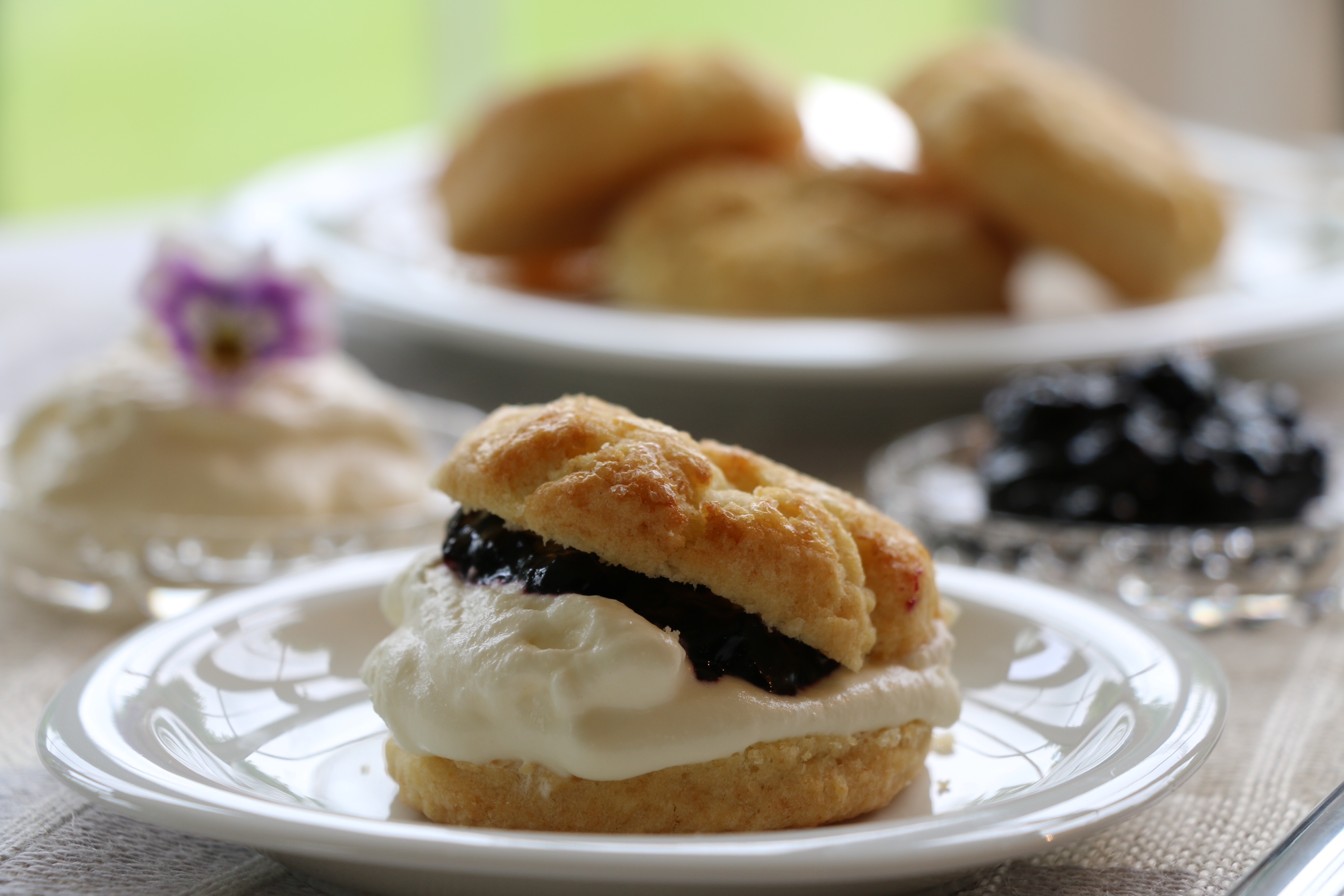This image captures an elegantly set table, possibly for a brunch or high tea. The focal point is a meticulously prepared scone, halved and filled with a generous layer of whipped cream and a dollop of dark berry jelly, sandwiched neatly on a white porcelain plate. This plate sits atop a textured fabric—perhaps a tablecloth or place mat. Adding to the refined presentation, a small flower adorns the top of the scone. Adjacent to the main plate, two clear glass dishes are visible, one holding additional berries and the other containing more cream. In the background, slightly out of focus, there is a bigger white porcelain plate holding several more scones or biscuits, hinting at a delightful spread. The entire setting suggests a sophisticated and inviting atmosphere, perfect for a special meal.